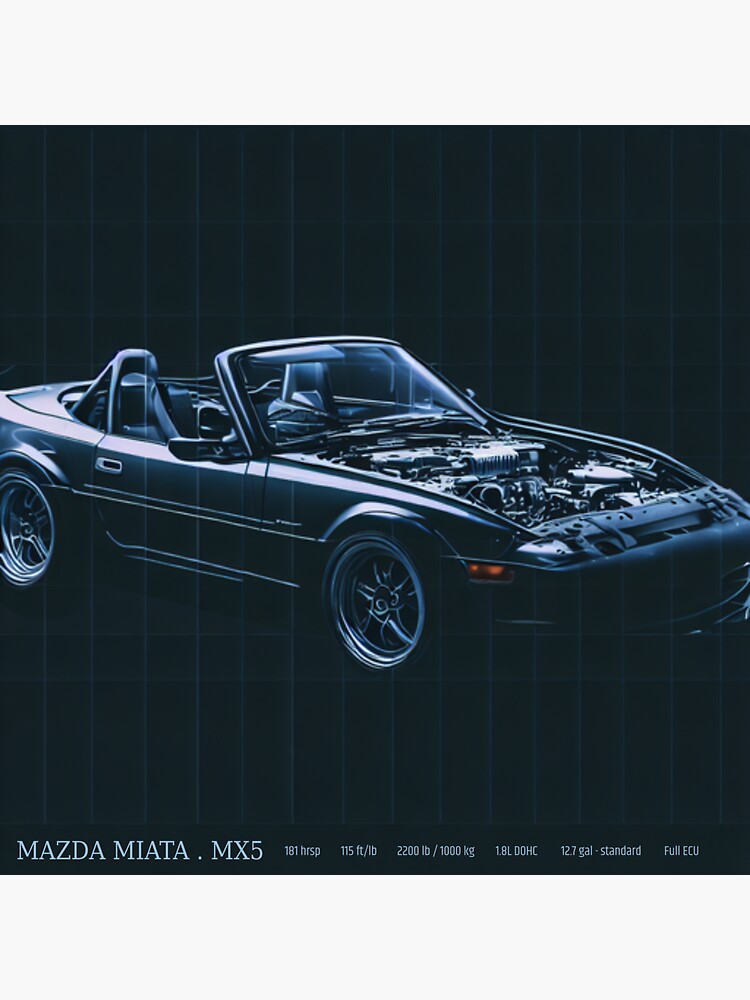This image features a detailed, diagrammatic portrayal of a Mazda Miata, with an almost monochromatic black and navy color scheme. The background is a subtle navy blue adorned with faint vertical and horizontal stripes. Positioned at the bottom in white text, it reads "Mazda Miata MX-5" followed by key specifications including "181 horsepower, 115 foot-pounds, 220 pounds/1000 kilograms, 1.8 DOHC, 12.7-gallon standard, full ECU." 

The car itself is depicted in the same navy hue as the background, highlighted with strategic lighting that accentuates its shiny spokes, tire rims, and the curvatures of its body. Uniquely, the front hood is absent, revealing an intricate view of the vehicle's internal mechanics. The convertible's clean windshield and the absence of a roof showcase the sporty interior, including the two front seats, emphasizing its sleek, open-top design. This captivating illustration exudes the essence of a compact, high-performance sports car.